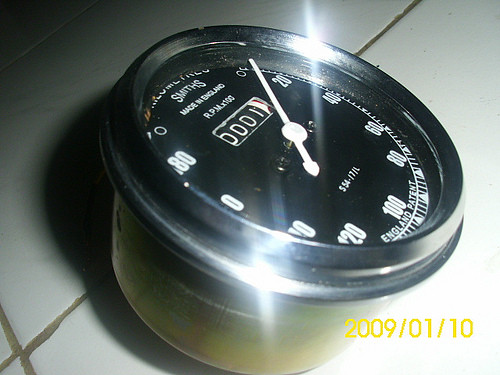This close-up photograph features a vintage black speedometer removed from a vehicle and placed on a white tiled floor with dark greyish-brown grout. The speedometer, angled slightly towards the camera, shows white numerals starting from 0 and increasing by increments of 20 up to 120. Due to the angle, the numbers on the left side are partially obscured by the speedometer's rim. The white pointer is positioned between the 0 and 20 marks.

In the center of the speedometer's face is a rectangular odometer displaying "0001". Above the odometer, "Smith's, Made in England, RPMX100" is inscribed in white text. The bottom right corner of the image shows a yellow date stamp "2009/01/10". The photograph also captures a shadow at the top left and a harsh shadow beneath the speedometer, likely caused by a camera flash, along with some glare on the speedometer's glass surface.